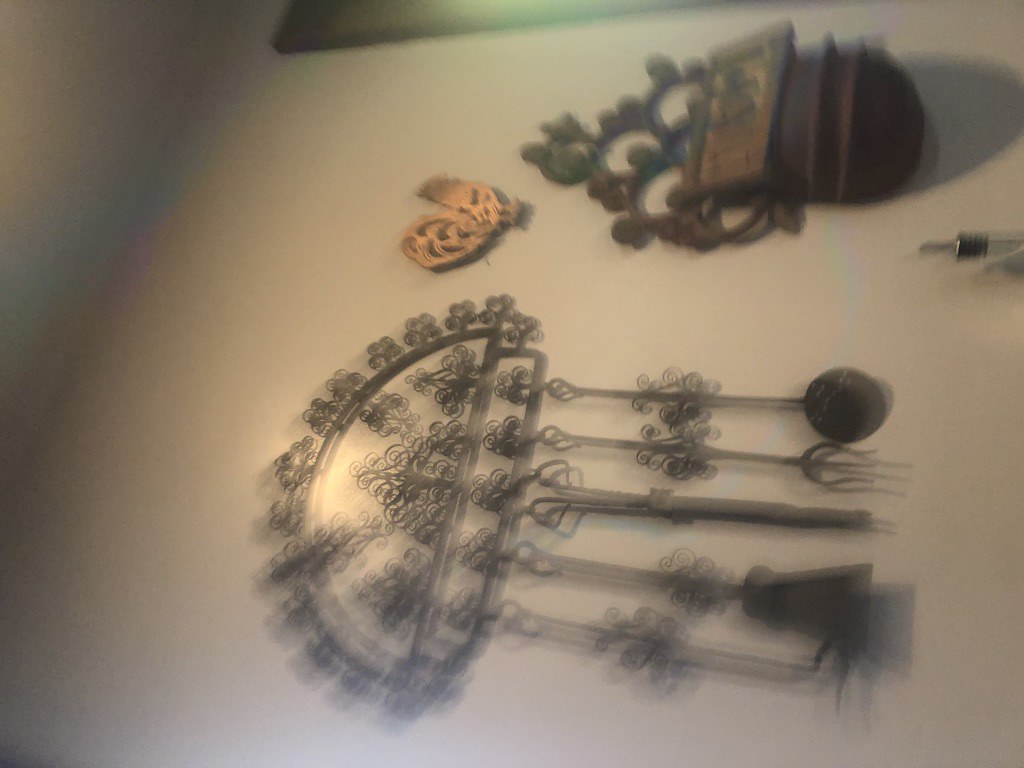This is a very blurry, sideways picture of a white wall adorned with various decorative items. The top of the image is actually the left side, and the bottom is on the right. The most prominent feature is a cast iron fireplace set hanging from a hanger shaped like a semi-circle with intricate swirly designs resembling trees or flames. This set includes multiple fireplace tools: a poker, a shovel, a pair of tongs, and a scoop, all hanging from long, decorative rods. To the right of the fireplace set, there's a noticeable bronze or gold metal carving of a rooster. Beneath this carving is a bulky wooden decorative piece with some unreadable text due to the blurriness. A door frame is faintly visible at the edge of the image.